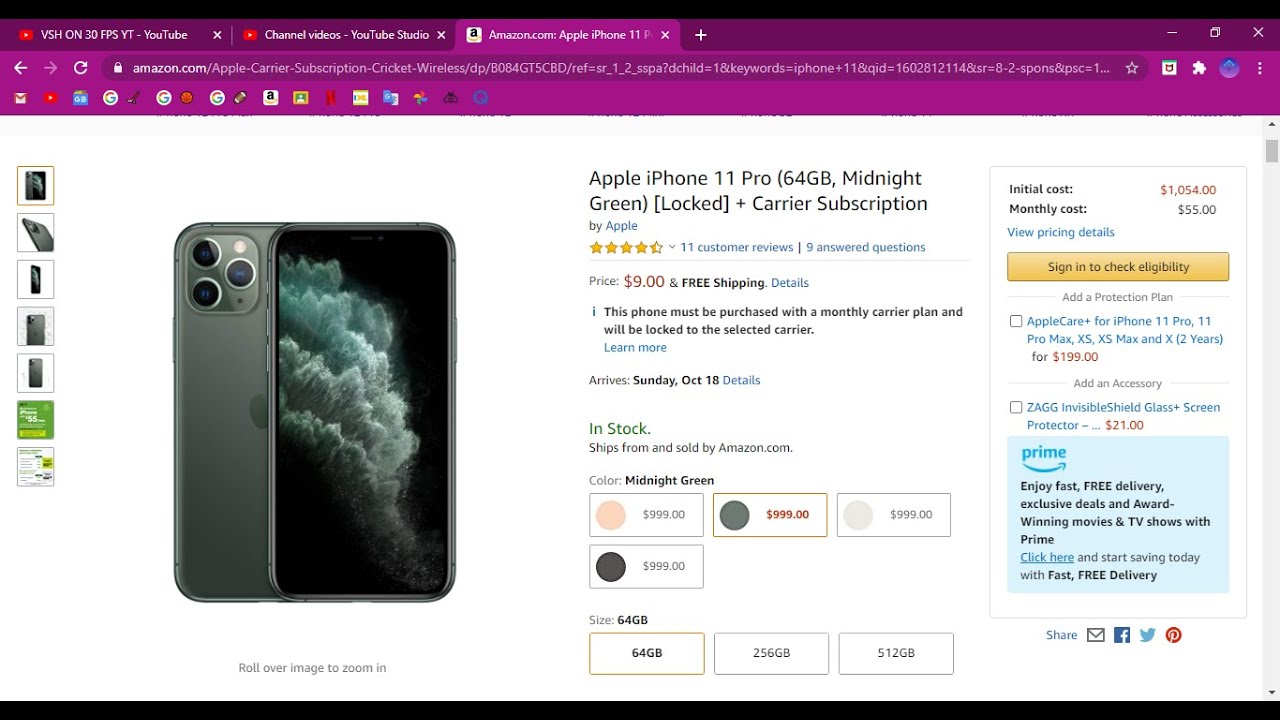In this detailed image, an Amazon Prime page is displayed, showcasing a search for an Apple iPhone 11 Pro. The prominently featured product is an Apple iPhone 11 Pro with 64GB of storage, in the color Midnight Green. The item is listed as locked and requires a carrier subscription. The product has garnered 11 customer reviews and boasts an average rating of four and a half out of five stars. 

The price is remarkably set at $9, accompanied by free shipping, although the total initial cost of the device is $1,054 with a monthly carrier plan of $55. The device will be locked to the chosen carrier and must be purchased with a monthly carrier plan.

The delivery date is noted as Sunday, October 10th, and the availability status is highlighted in green, indicating that it is in stock, sold by and ships from Amazon.com. The listed color is Midnight Green, with additional color options represented by circles: Pink, Green, White, and Black. Storage options include 64GB, 256GB, and 512GB.

A section invites customers to sign in to check their eligibility. There's also an option to add AppleCare for the iPhone 11 Pro, and the opportunity to purchase a ZAGG InvisibleShield glass screen protector for $21. 

A blue Prime badge in the left-hand corner indicates that fast, free delivery is available for Prime members.